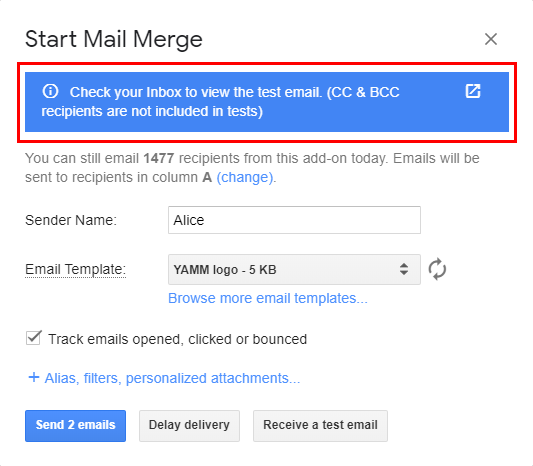The screenshot depicts a user interface for initiating a mail merge using an add-on. At the top of the page, a notification indicates that the action needed is to start the mail merge. Users are instructed to check their inbox to view the test email. It clarifies that CC (Carbon Copy) and VCC (Blind Carbon Copy) recipients are not included in the test emails. The interface informs the user that they have the capacity to send emails to 1,477 recipients using this add-on today, targeting recipients listed in column A of a spreadsheet. There is an option labeled "change" for users who wish to alter which column the emails are sent to.

The sender is named, and an email template titled "YMM logo" is specified, with a file size of 5 kilobytes. Below this, there is a checkbox option to "track emails opened, clicked, or bounced," which is currently selected. Additional options are provided for adding alias filters and personalized attachments.

At the bottom of the interface, there are several buttons: one in blue labeled "send two emails" and others in gray labeled "delay delivery" and "receive a test email." This indicates that the user is in the process of setting up a mass email campaign, possibly in the testing phase rather than ready for full deployment. The background of the interface is a simple and clean white.